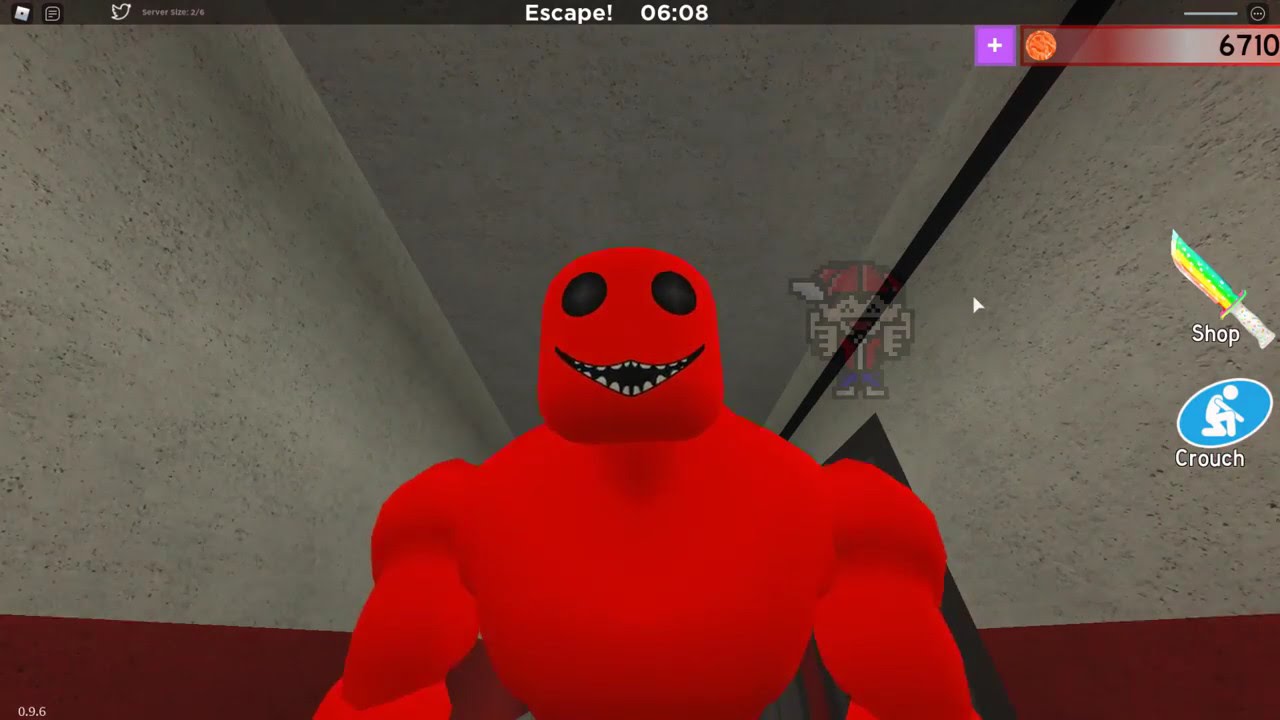This image appears to be a screenshot from a video game with cartoonish graphics, possibly a horror-themed game. Dominating the center is a red, muscular, monster-like character with smooth, rounded rectangle-shaped head, large black eyes, and a wide, black smile displaying sharp white teeth. The character is set against a backdrop of gray cement walls with a red stripe running along the bottom and a gray cement ceiling. A ghostly, pixelated boy wearing a red hat and shirt with blue pants hovers just above the character's left shoulder, adding to the eerie atmosphere.

On the right side of the screen, a rainbow-colored knife icon labeled "Shop" and a blue and white crouching figure labeled "Crouch" are prominently displayed. The top of the image features a black horizontal border with social media icons on the left, the word "Escape!" in white text in the center, and a timer reading "06:08" next to it. In the upper right corner of the screen, the number "6710" likely indicates a score, accompanied by an icon that resembles a coin or fireball. This detailed setup suggests various game elements, contributing to the immersive gaming experience.